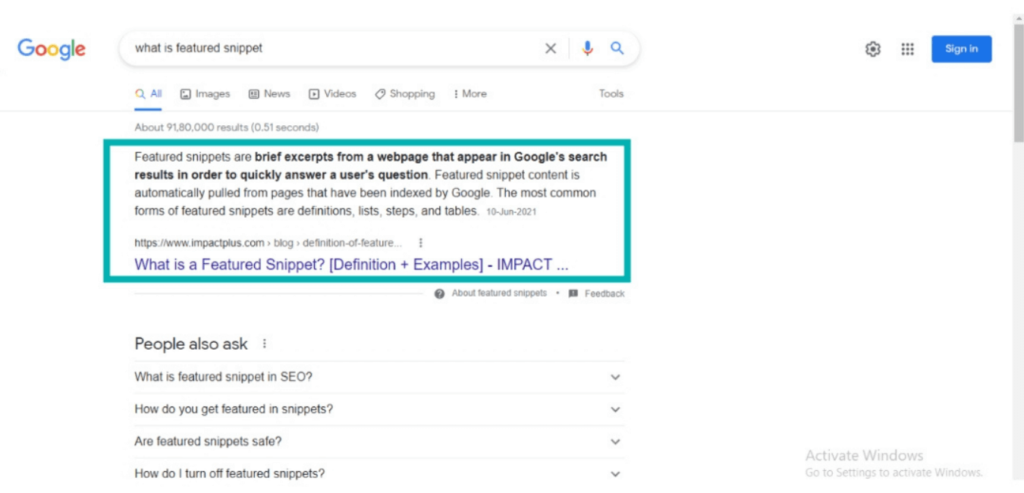This detailed screenshot captures a Google search results page showing a query about "featured snippet." The search bar, adorned with the Google logo on the left, displays the user's input query: "what is a featured snippet." To the right of the search bar are an "X" icon, a microphone icon, and a magnifying glass icon representing the search function.

Below the search bar, there are multiple navigation tabs: "All," "Images," "News," "Videos," "Shopping," "More," and "Tools," with "All" being actively selected—indicated by its blue color and underlining. The results count shows approximately 9,180,000 results generated in 0.51 seconds.

Prominently highlighted within a teal box is a featured snippet that reads: "Featured snippets are brief excerpts from a web page that appear in Google search results in order to quickly answer a user's question. Featured snippet content is automatically pulled from pages that have been indexed by Google. The most common forms of featured snippets are definitions, lists, steps, and tables." The snippet content is cited from 10 June 2021.

Following the snippet, the original query "what is a featured snippet" is displayed again in purple. Below this, there is a "People also ask" section with related questions such as "What is a featured snippet in SEO?", "How do you get featured in snippets?", "Are featured snippets safe?", and "How do I turn off snippets?". Each question has a clickable drop-down arrow for further details.

At the bottom of the featured box, there are links labeled "About featured snippets" and "Feedback."